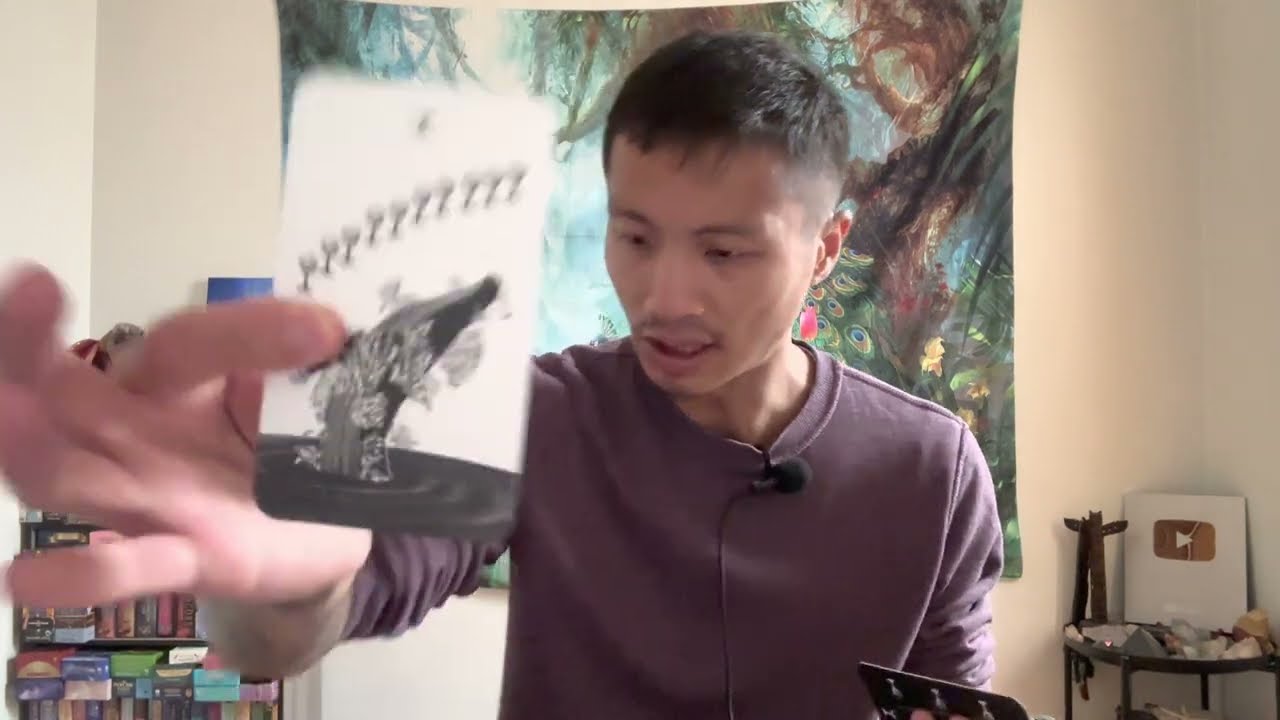The photograph portrays a young man, possibly of Asian descent, sitting in front of a camera, suggesting he is likely a YouTuber. He has dark hair and a mustache, and he wears a purple long sleeve shirt with its arms pushed up above his elbows. Attached to the collar of his shirt is a black microphone. The man is holding up a black and white playing card with a whale breaching from the water in his right hand, while his left hand holds another playing card. Behind him, a colorful tapestry featuring vivid peacock-like feathers spans the wall. To the side of the room, there is a round table displaying a YouTube award, accompanied by a black statue and an array of crystals and rocks underneath. Opposite the tapestry are various multicolored boxes in shades of purple, pink, blue, black, and red, adding a lively touch to the white room. The overall scene is one of a content creator possibly engaged in a magic trick or an unboxing haul video, captured from a perspective that might be from a laptop screen.